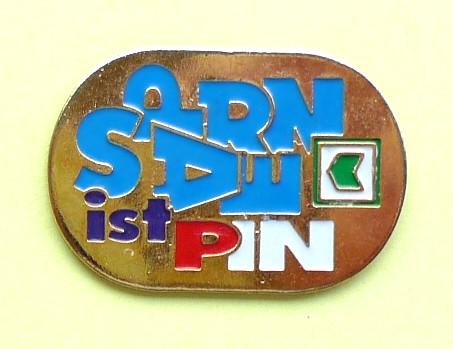This photograph features a metallic, oblong or lozenge-shaped pin set against a yellow background. The pin has a gold-hued base and is adorned with a series of jumbled letters and a symbol, all in various colors and fonts. At the top of the pin, the letters are arranged vertically and sideways, spelling "S-P-A-R-E-N" in shades of blue. To the right of this lettering, there is a square with a green border enclosing a white field, within which a green arrow points to the left. Below the blue letters, additional characters spell out "I-S-T" in purple. The word "PIN" follows, with the "P" in red and the "I-N" in white. The combination of vibrant colors and the unique arrangement of symbols makes the exact wording somewhat difficult to decipher, but the overall design is eye-catching and detailed.